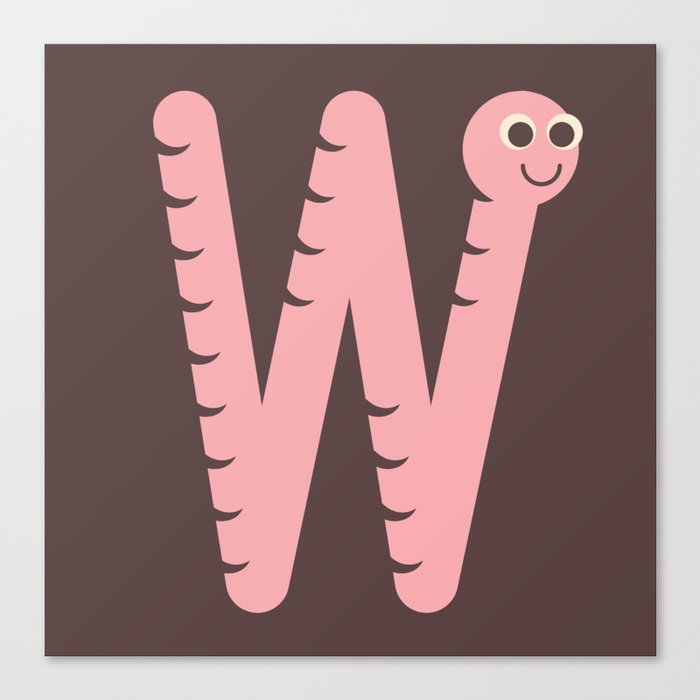The image is a digital graphic illustration of a pink worm, intricately detailed and whimsically designed to form the shape of the letter "W". This captivating worm has numerous dagger-like, triangular brown stripes running the length of its body, reminiscent of tiger stripes. At the top right end of the "W", the worm features a circular head with large, expressive googly eyes—each eye is white with a large black pupil. A small, playful crescent forms the worm's smiling mouth. This endearing character is placed at the center of a purplish-brown square, which is itself framed by a very light gray background, giving an impression of a picture frame or logo.